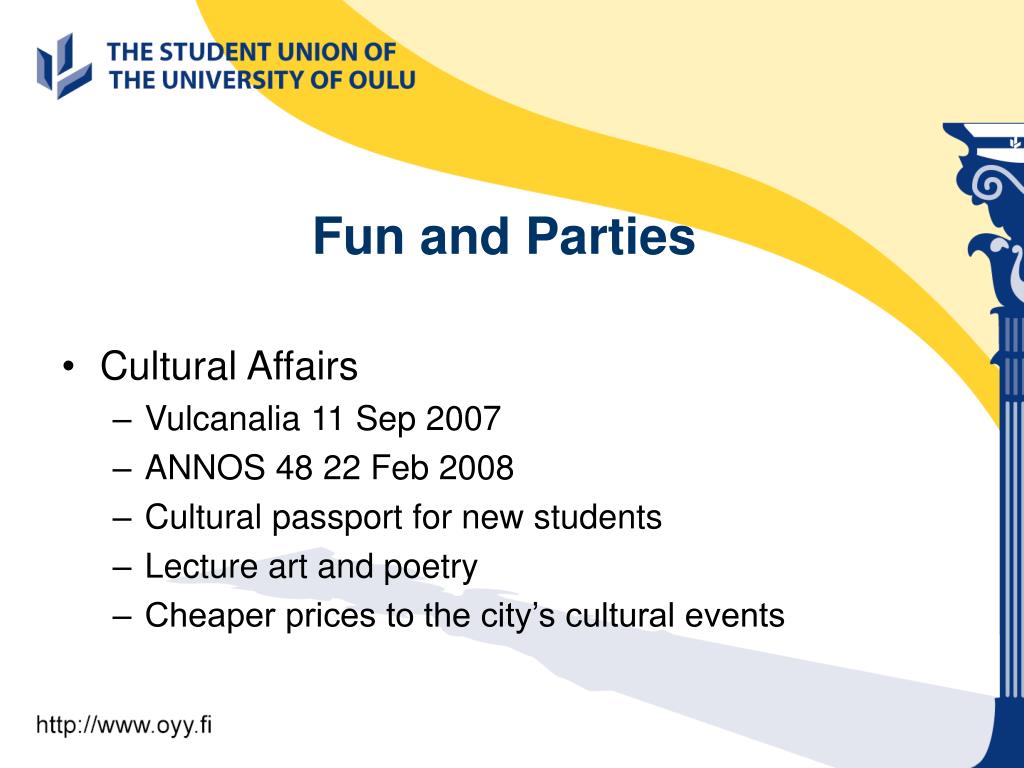This image appears to be an online brochure or PowerPoint slide from the Student Union of the University of Oulu, prominently titled "Fun and Parties." In the upper left corner, the text "Student Union of the University of Oulu" is displayed in blue, accompanied by the university's logo featuring blue shapes. A light creamy butter yellow area occupies the top right, with a brighter yellow streak just below it. To the far right, there's a blue depiction of a Roman column. The main content includes bullet points listing:

- Cultural Affairs
- Vulcanalia, 11th September 2007
- ANNOS, 22nd February 2008
- Cultural Passport for New Students
- Lecture, Art, and Poetry
- Cheaper Prices to the City's Cultural Events

Additionally, the lower left corner provides a website link: http://www.oyy.fi.